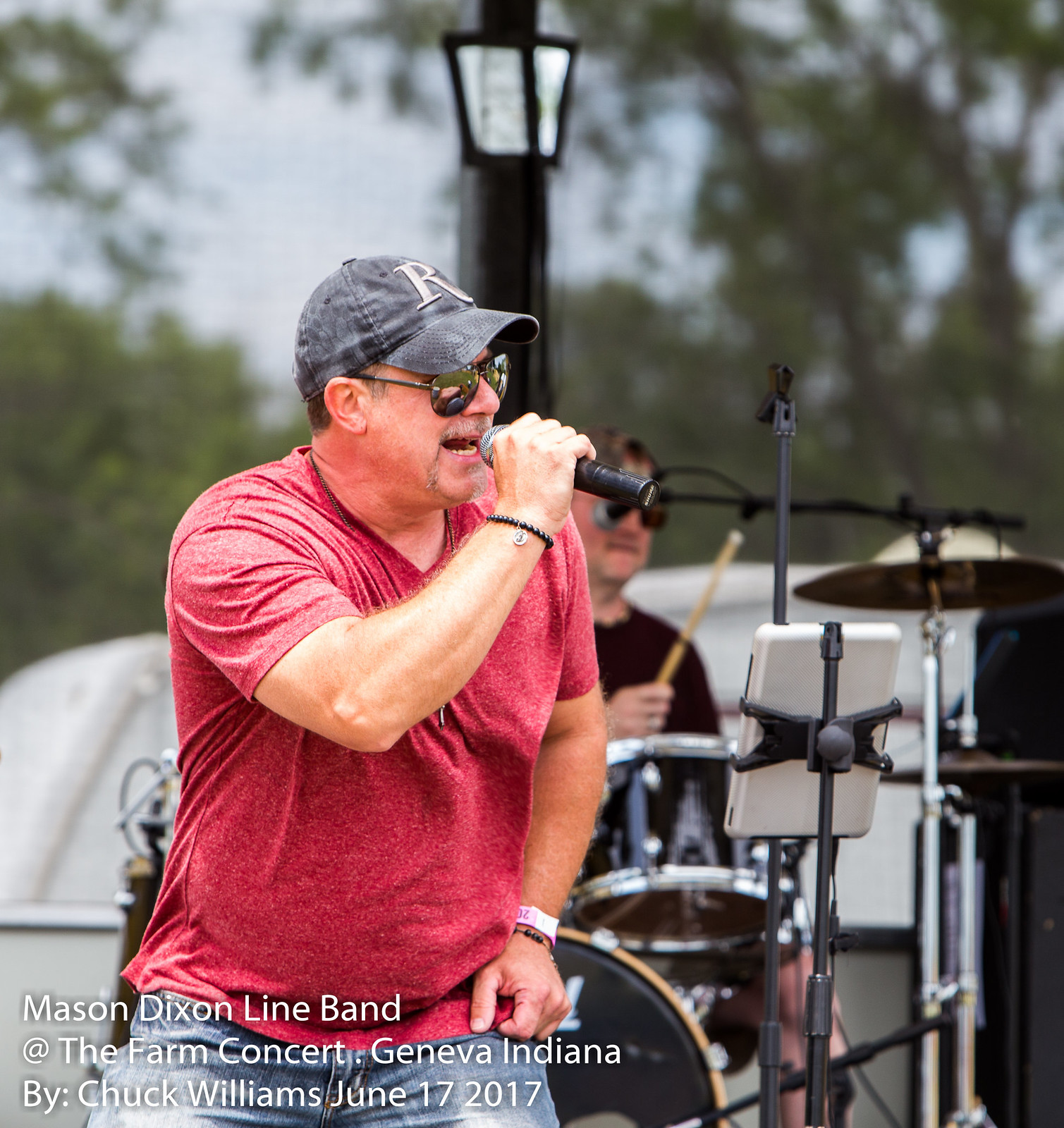The image captures an outdoor concert of the Mason Dixon Line Band at the Farm Concert, Geneva, Indiana on June 17, 2017, taken by Chuck Williams. The main focus is on an older, heavy-set Caucasian singer who is holding a microphone up to his mouth. He sports a blue cap with a capital letter 'R', sunglasses, a gray mustache, and a reddish-pink t-shirt. He also wears a bead bracelet with something hanging off it and blue jeans. The blurred background shows trees, the sky, and a light pole. Behind the singer, another Caucasian man is visible, partially obscured, playing the drums while wearing sunglasses and a black shirt. The stage is set for a vibrant outdoor performance under a sunny sky, emphasizing the lively atmosphere of the event. The lower left corner of the image is labeled "Mason Dixon Line Band at the Farm Concert, Geneva, Indiana by Chuck Williams, June 17, 2017."